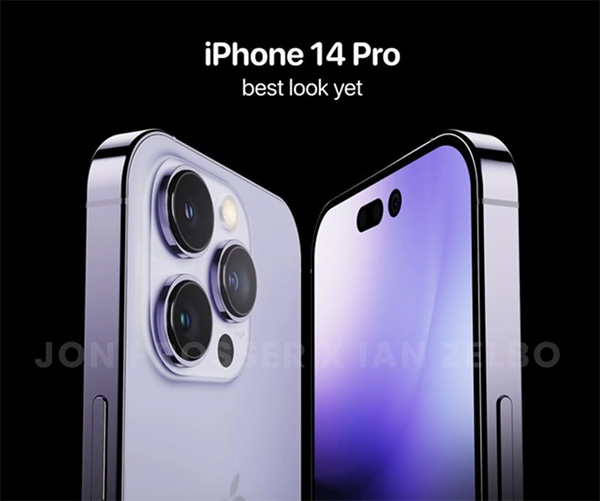A high-resolution advertisement showcases the iPhone 14 Pro against a stark black background, accentuating its sleek, modern design. The image features the top half of the phone's back, prominently displaying its three advanced camera lenses and the side button, enhanced by a monochrome color scheme that exudes sophistication. On the right side of the ad, the front of the iPhone is depicted with a blank, subtly purple screen. A watermark, though indistinct, overlays the entire image.

The caption "iPhone 14 Pro: Best Look Yet" is boldly written in white at the top, emphasizing the phone's superior design. Below, a secondary line centrally affirms, "Bigger and Bolder," reinforcing the iPhone 14 Pro's commanding presence. This minimalist advertisement focuses solely on the visual appeal of the iPhone 14 Pro, declaring it as their best-looking model to date with unparalleled aesthetic excellence.